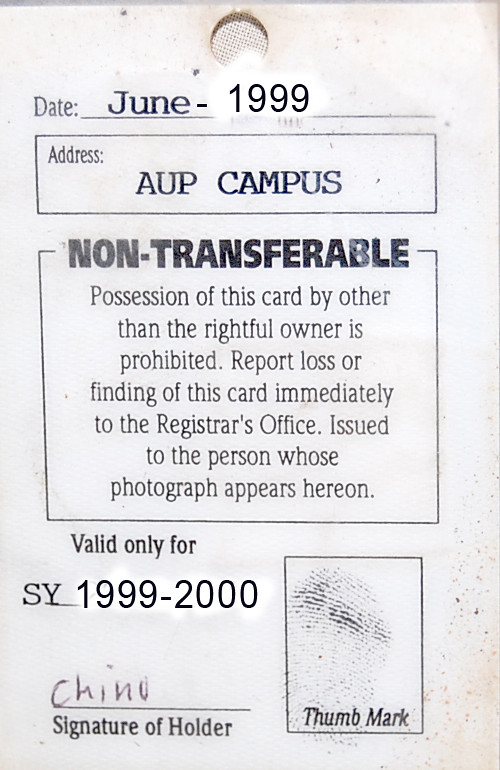This image features a white poster or card, which appears to be a student-related identification or access pass dated June 1999. The card includes black text and numerous details pertinent to its function and owner. At the top, there’s a cut-out circle, possibly indicating it was intended to be hung. The text specifies it is non-transferable, and possession by anyone other than the rightful owner is prohibited. It must be reported to the Registrar's Office if found. The card is valid only for the academic year 1999 to 2000 and is issued to a student named Chino, whose signature appears at the bottom. Additionally, there is a designated area for a thumb mark on the bottom right, which contains a visible thumbprint, confirming the card's validity for the respective student. The address 'AUP Campus' is also noted, further indicating its likely association with a university or college.